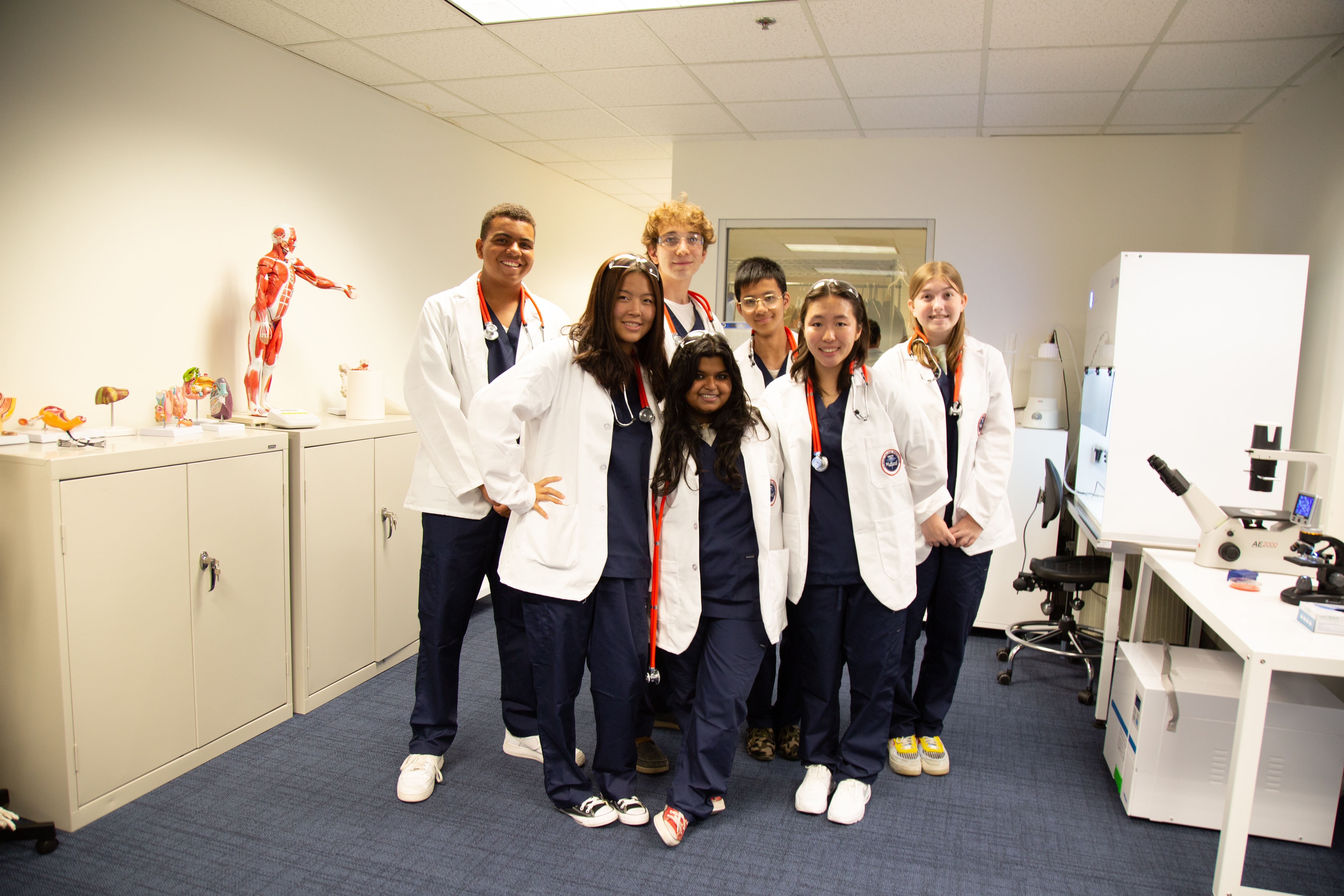The image depicts a group of seven individuals, likely young medical trainees or new doctors, standing in the center of a white-walled lab with a bluish carpet. The group consists of four women in the front row and three men in the back row, all wearing white lab coats over dark blue scrubs, with stethoscopes around their necks. Their faces are lit with smiles, suggesting a positive and lighthearted moment. 

To the left side of the room stand two beige metal cabinets. Atop these cabinets rest anatomical models, including a red and white human body model and various plastic organ models like the liver. On the right side, a white table supports a microscope along with other testing equipment. The ceiling features multiple square panels, indicating a functional and well-lit environment. The overall composition seems to hint at a class photo or a field trip, where the young participants are possibly exploring medical science.